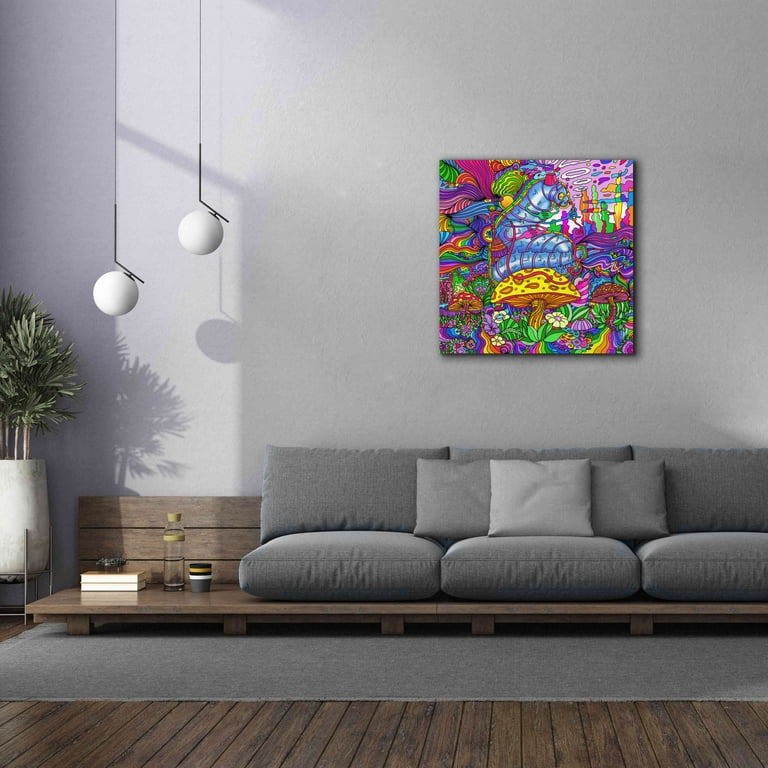The image depicts a modern living room with a distinct focal point on a unique, low-to-the-ground wooden couch. This couch features removable brown cushions and gray throw pillows, and extends to the left to form an integrated end table adorned with books and cups. The couch sits on a gray rug that contrasts with the dark brown plank flooring. Above the couch, a vibrant, psychedelic painting captures attention with its explosion of colors, including reds, yellows, greens, pinks, blues, and oranges. The artwork depicts a whimsical scene with a yellow mushroom, wavy lines, clouds, flowers, and more, all contributing to its vivid and striking appearance. The room’s light gray walls enhance the painting's vibrancy, making it stand out as the main focal point. Natural light floods the room, supplemented by two circular ceiling lights above the end table, creating a bright and inviting atmosphere. A green potted plant on the left side adds a touch of nature to the modern setting.